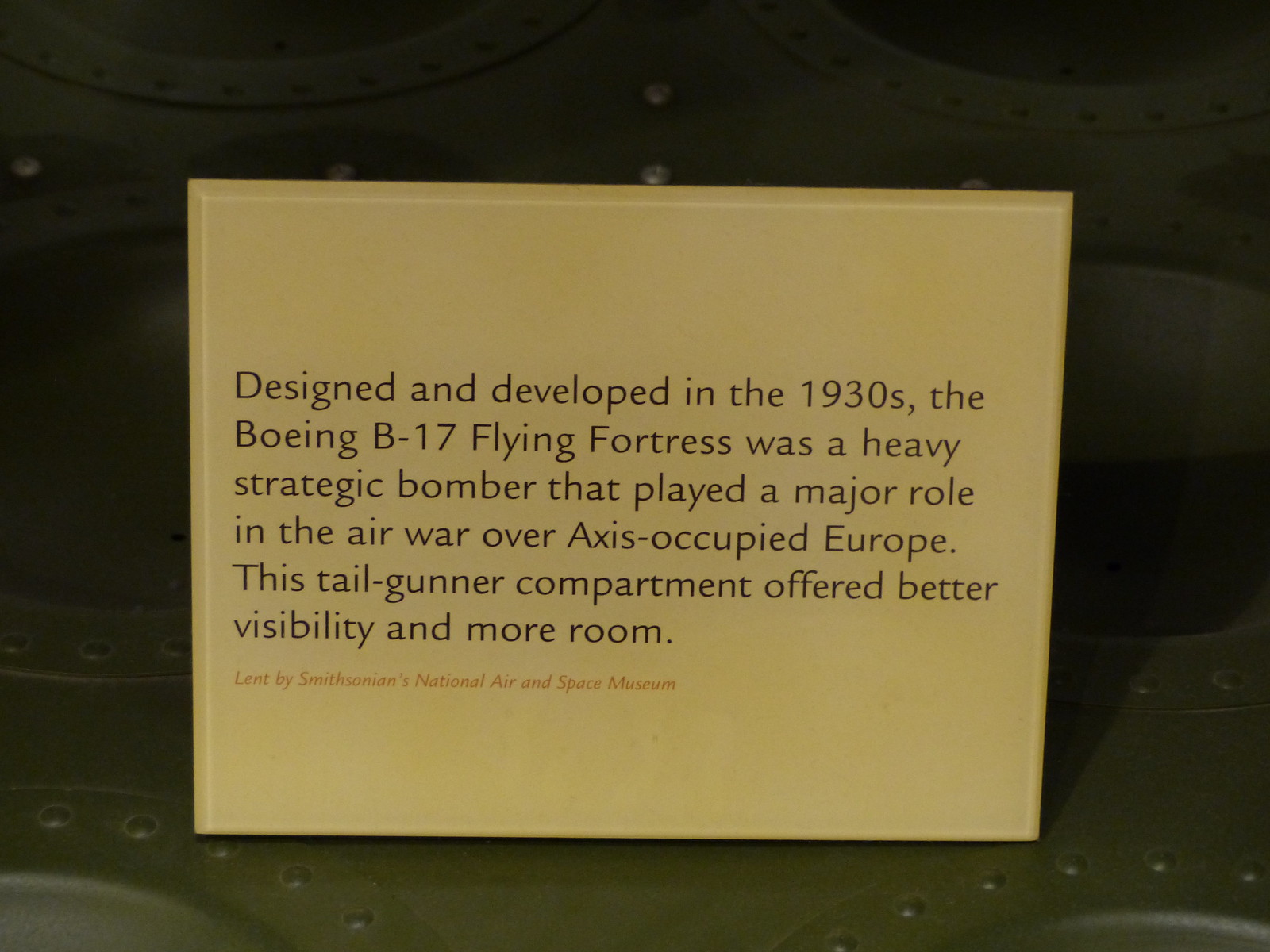The image features a sign or explanation card with a yellow background and black text that reads: "Designed and developed in the 1930s, the Boeing B-17 Flying Fortress was a heavy strategic bomber that played a major role in the air war over Axis-occupied Europe. This tail gunner compartment offered better visibility and more room." Below this, there is a footnote in small orange text stating, "Lent by Smithsonian's National Air and Space Museum." The sign is set against a backdrop of dark green metal, which appears to be part of a large machine. The dark green metal is adorned with circular arrangements of rivets, adding to the industrial aesthetic. The overall scene suggests the sign is likely in a museum exhibit, perhaps in front of the actual tail gunner compartment of a Boeing B-17 Flying Fortress.